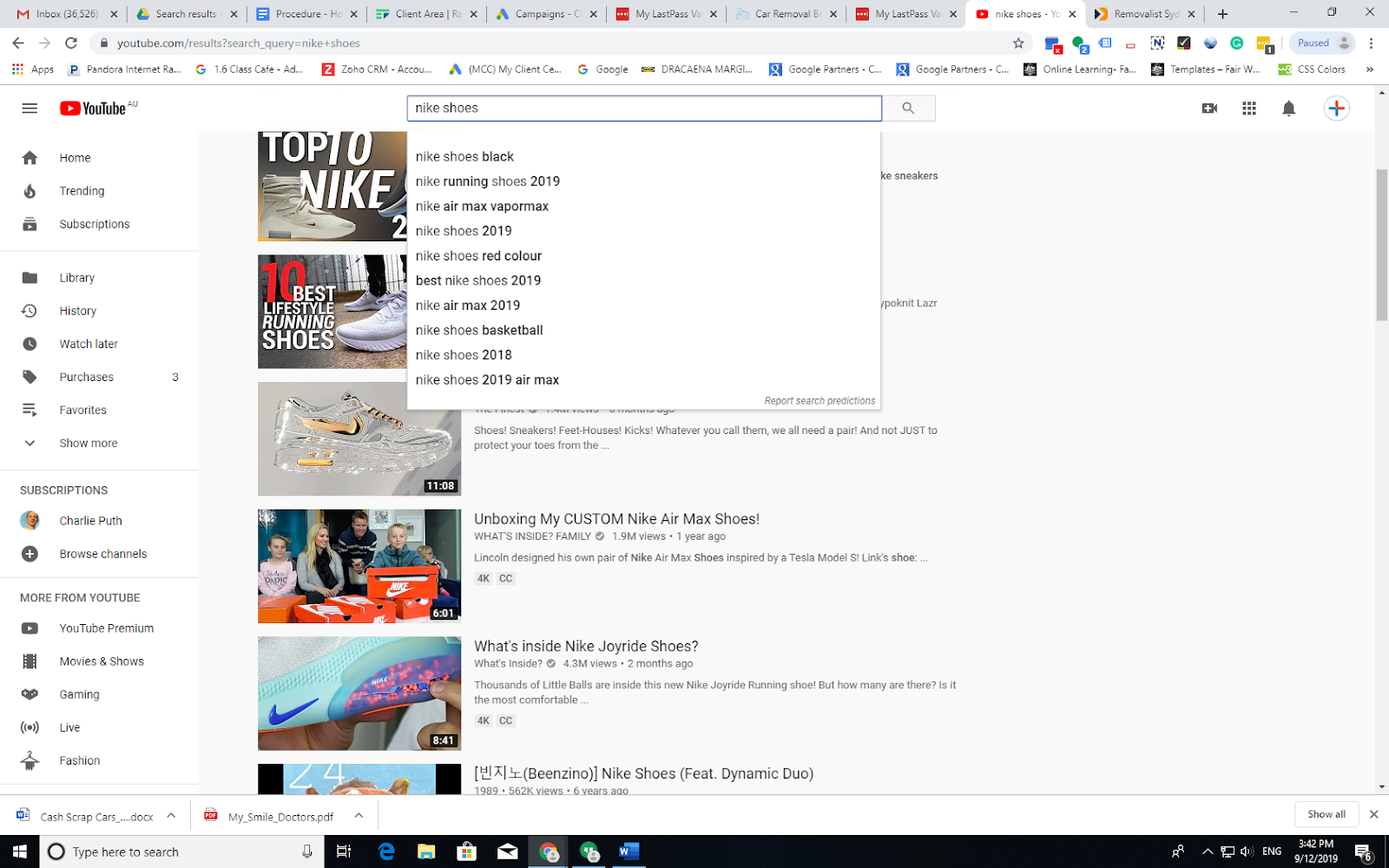The image displays a YouTube search results page for the query "Nike shoes." The URL at the top suggests it is a results page, although the full address is partially obscured. In the center of the screen, "Nike shoes" is prominently displayed as the search term. Below it, multiple search results are listed, including:

- Nike shoes black
- Nike running shoes 2019
- Nike Air Max
- Vapor Max
- Nike shoes 2019
- Nike shoes red color
- Best Nike shoes 2019
- Nike Air Max 2019

Each of these search terms is accompanied by clickable video thumbnails. The thumbnails show various visual representations and styles of Nike shoes, but one in particular stands out as it appears to feature a clear, possibly crystal shoe, suggesting a decorative item rather than a functional piece of footwear. Among the thumbnails, the sixth result appears partially visible and includes the name "Benzino" alongside an unclear section of Korean text.